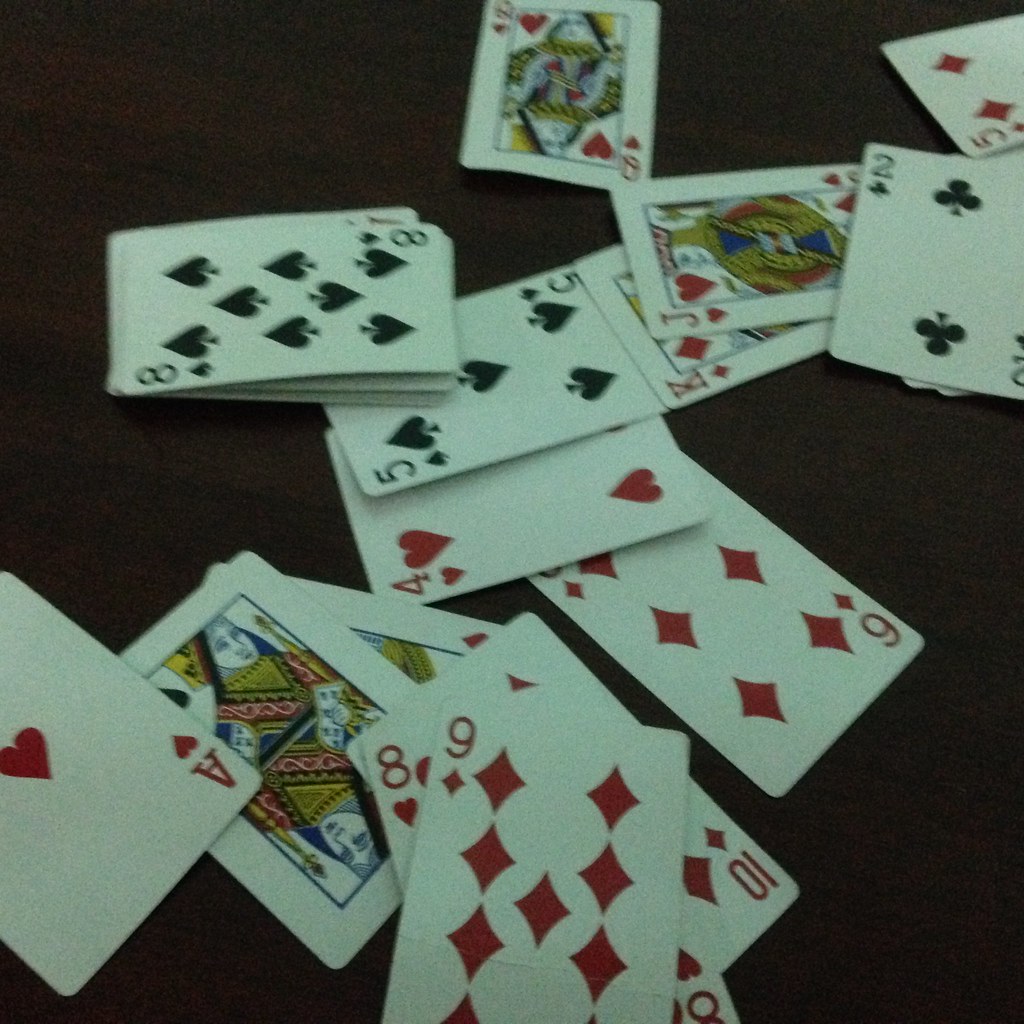In this photograph taken by an unknown photographer, a collection of playing cards lies scattered across a dark, brownish surface that remains indistinct, potentially a table, floor, or carpet. The cards visible face-up include: the 9 of Diamonds, 8 of Hearts, 10 of Diamonds, Queen of Spades, Ace of Hearts, Queen of Diamonds (partially obscured), 6 of Diamonds, 4 of Hearts, 5 of Spades, 8 of Spades, Queen of Hearts, Jack of Hearts, King of Diamonds, 2 of Clubs, and the 5 of Diamonds. Additional cards are present underneath these but are not visible. The arrangement showcases both red and black suits, adding a classic contrast to the image. No other significant elements or subtleties are apparent in the composition.